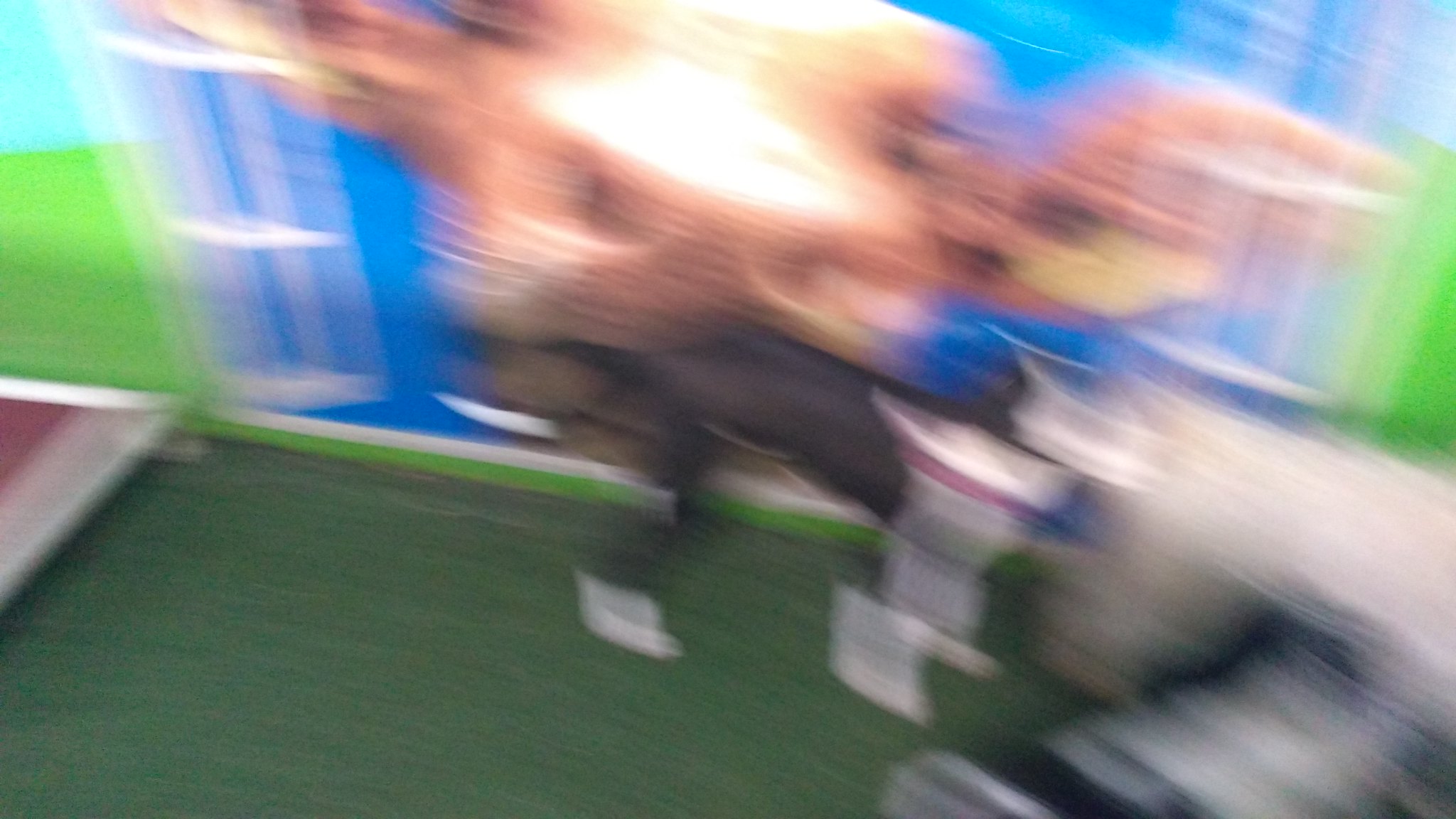In this blurry yet vibrant photograph, a black and white dog stands prominently on a patch of astroturf, positioned centrally within the frame. The dog’s chest, front legs, and parts of its head are white, contrasting sharply with its mostly black back and hind legs. A red collar adorns its neck, adding a pop of color. Behind the dog, the background is dominated by a large, blue-tinged screen featuring the image of a cow's face looking directly at the viewer, its ears jutting out on either side. The scene is further cluttered by an indistinct, blurry black and white object on the right and another unclear, white object in front of the dog. Despite the overall blurriness, the photo exudes a colorful and lively ambiance.